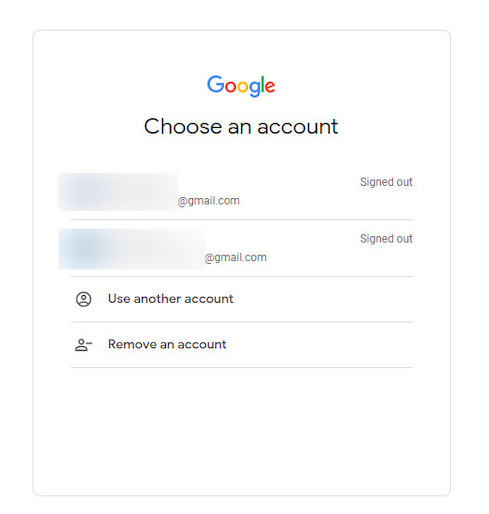The image is a simple screenshot showcasing a section of Google's login interface. At the very top of the screenshot, the Google logo is prominently displayed, featuring its iconic multi-colored design. The logo consists of a capital "G" in blue, followed by a lowercase "o" in red, another lowercase "o" in yellow, a lowercase "g" in blue, a lowercase "l" in green, and a lowercase "e" in red.

Beneath the logo, the text instructs users to "Choose an account." Two email addresses are partially visible, both ending with "@gmail.com." The initial sections of these email addresses are obscured by a blue box, concealing the full addresses. Next to each email address, there is a corresponding button; the first email has a "Sign up" button on its right, while the second, longer email address has a "Sign out" button on its right.

Below the listed accounts, a horizontal line separates additional options. Users are prompted to "Use another account," accompanied by a grey circular icon depicting a head and shoulders silhouette.

Further down, the option to "Remove an account" is presented, featuring an icon of a head and shoulders silhouette with a minus sign adjacent to it. The entire interface is set against a clean, white background with text in black and dark blue, creating a clear and user-friendly visual.